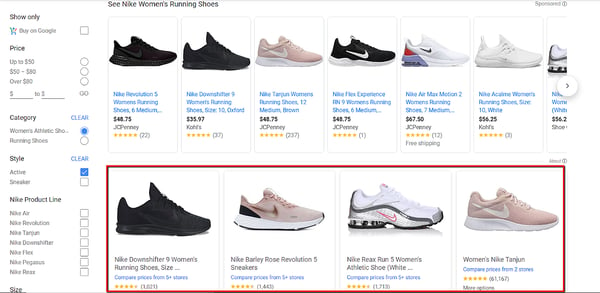Screenshot of a Retail Website Featuring Nike Women's Running Shoes:

This image captures a screenshot from a retail website dedicated to selling shoes, prominently featuring Nike women's running shoes. Near the upper left corner of the screenshot, a heading reads, "See Nike Women's Running Shoes."

The page displays two rows of Nike sneakers, each accompanied by detailed descriptions and ratings. 

One of the sneakers, positioned third from the left in the top row, is pink and white. Below this shoe, the caption reads: "Nike Targon Women's Running Shoes, 12 Medium Brown, $48.75 at JCPenney." This sneaker has received a high rating of five stars from 237 reviewers.

Another sneaker in the top row is all white. Its description states: "Nike Arcane Women's Running Shoes, Size 10 White, $56.25 at Kohl's." This shoe has garnered approximately 35 five-star ratings.

In the bottom row, the leftmost sneaker is entirely black. The caption underneath it conveys, "Compare prices from five stores." It appears that the user clicked on the bottom row, likely to see the price comparison for this particular black sneaker.

The screenshot provides a clear view of the sneakers, their prices, specific retailers, and customer ratings, offering a detailed snapshot of available options for Nike women's running shoes.